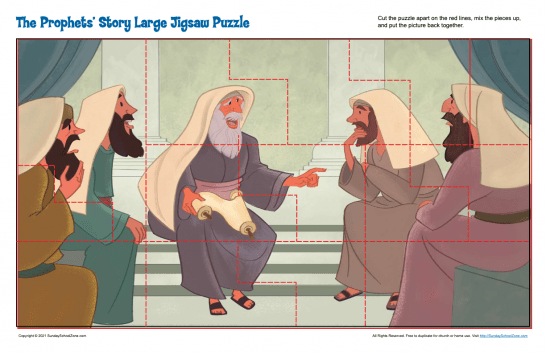This is a detailed depiction of a colorful rectangular jigsaw puzzle titled "The Prophet Story Large Jigsaw Puzzle." The puzzle’s instructions, written in small black font, advise cutting along the red dotted lines marked throughout the image to disassemble and reassemble the pieces. The central image shows five men, all with beards, seated on concrete steps in front of a marble building, engaged in conversation. In the middle, an elderly man with an all-white, long beard and wearing a robe and sandals, points to a man beside him who has a brown beard and strokes it pensively. The men are dressed in robes and head coverings, with the remaining individuals featuring various beard colors, including black and brown. The scene vividly captures a thoughtful moment of discourse among the men, framed by the puzzle's red lines and set within the context of ancient times.